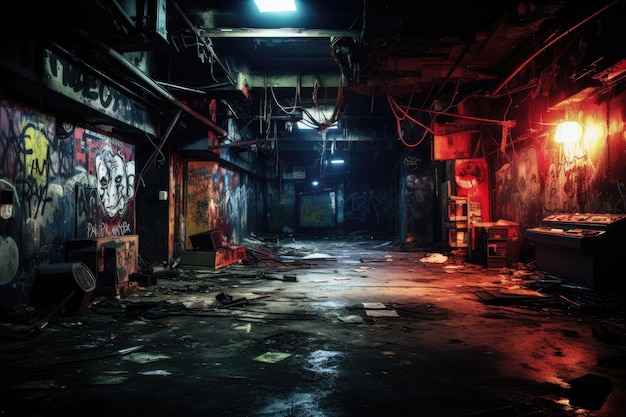The photograph showcases an old, abandoned factory that exudes an eerie, basement-like atmosphere. The expansive space features high ceilings, painted green, from which numerous wires and brown beams dangle precariously. The setting feels industrial and gritty, with floors littered with metal sheets, magazines, and general debris, all hinting at long-term neglect and disarray. The factory walls on both sides are covered with extensive graffiti, including a notable zombie-like face painted on the left wall. Despite the overall darkness, the image is punctuated by a few sources of light: a rectangular white lamp on the ceiling and a conspicuous bright yellow light mounted on the right wall, casting a grim illumination over the dilapidated environment, adding to the haunting mood of the abandoned space.